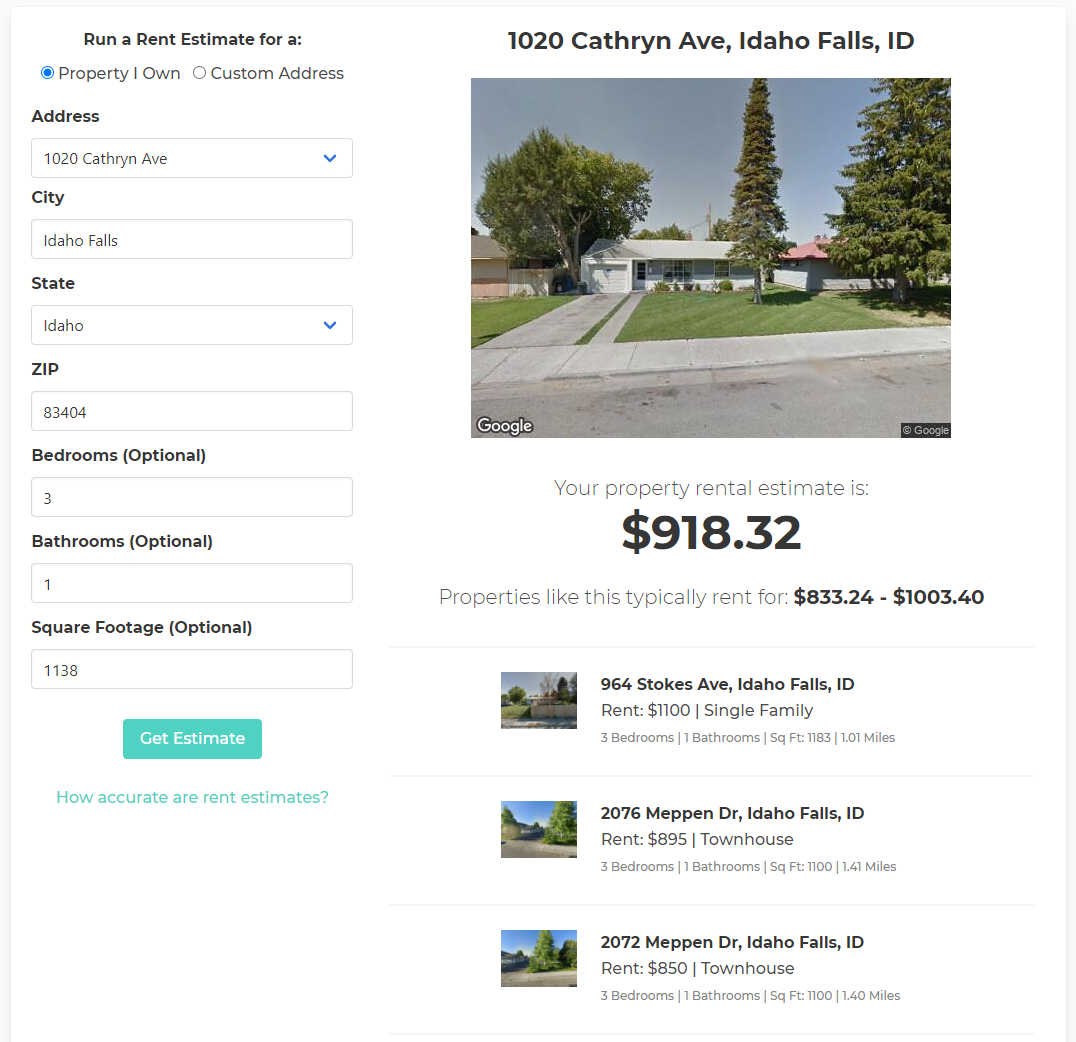The image depicts an individual using a website to list their property for rent. The website interface lacks a visible name, but it displays various property details and entry fields. On the left, the user has filled in information: property ownership, address, city, state, zip code, number of bedrooms and bathrooms, and the property's square footage. 

Based on this information, the site generates a rental estimate of $918.32 per month. Adjacent to this value, there is a range indicating that similar properties typically rent for between $833.24 and $1,003.40. Below this estimation, there are listings of comparable properties with their respective rental prices, offering a comparative analysis for the user.

From the photo included in the listing, it appears that the image was obtained using a Google tool, as indicated by the "Google" watermark present at the bottom corners of the picture. This suggests that the individual utilized a Google program to capture the required visual for their rental property listing. It seems the user is aiming to make a well-informed rental decision amid the current, less-than-favorable housing market conditions.